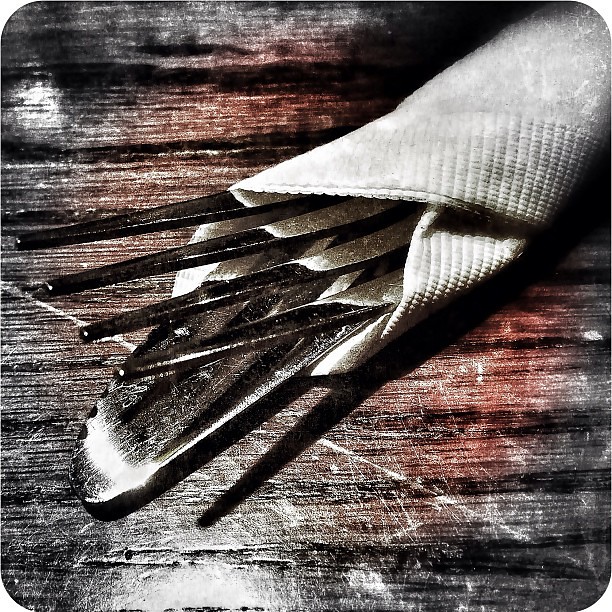This photograph, likely created digitally or with a photo editing tool, showcases a tightly framed, detailed close-up of silverware carefully wrapped in a napkin. The rich details of the reddish-brown wooden table fill the background, revealing a burgundy hue interspersed with white scratches and black horizontal indentations that highlight the texture and age of the surface. The silverware includes the tines of a silver fork—four in number—and the top edge of a silver butter knife, both of which catch and reflect the light. The cutlery is wrapped in a thick gray napkin, featuring a textured, square pattern at the top and a ridged border around the edges. The image captures the succinct setup with remarkable clarity, emphasizing both the metallic sheen of the utensils and the rustic charm of the worn wooden table beneath.